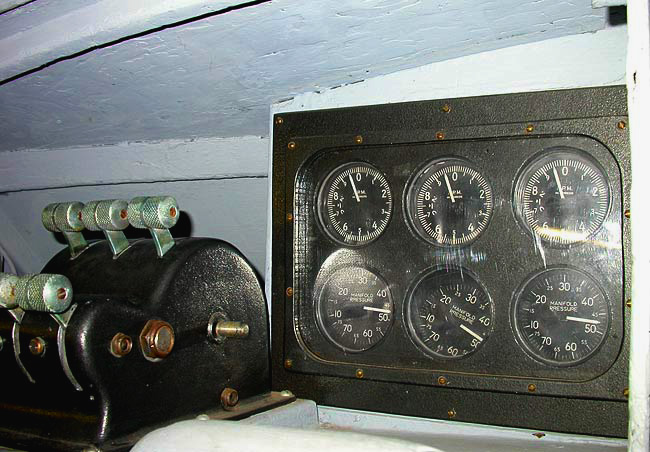An extremely detailed, close-up image captures a section of a wall-mounted machine. The wall itself is white with a noticeable texture. On the left side of the machine, there are six metal handles with a greenish hue, each accentuated by a rusty nail and textured grips, transitioning into a smooth surface in the middle part of the machine. To the right, embedded in the wall, is a black metal component featuring six thermometers, each displaying different readings. The thermometers have black and white markings and are secured by gold-colored nails. The image appears to have been taken with a flash, evident from the reflection on the black metal surface, which also shows minor scratches.